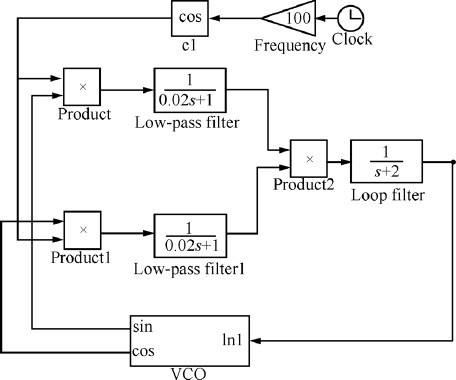This detailed diagram, rendered in black and white, represents an intricate flowchart that depicts the components of an electrical circuit, likely aiming to illustrate a mathematical model. Beginning at the top right corner, the diagram features a small, simple clock icon labeled "Clock." An arrow from the clock directs to a triangle marked with the number "100" and labeled "Frequency." Following the flow, the next component is a square with the notation "COS" under which "C1" is inscribed. This square’s arrow proceeds to multiple elements, including a labeled "Product" symbolized by an 'X,' followed by a rectangle marked "Low Pass Filter" with the equation "1/(0.02s + 1)" inside. 

Continuing along, another arrow leads to "Product 2," which also transitions into a "Loop Filter," characterized by the equation "1/(s+2)." The final component in the sequence is a rectangle labeled "VCO" ("n1"), containing sine and cosine notations, indicative of voltage-controlled oscillation. Other elements distributed throughout the flowchart include additional products and a second low pass filter, integrating various mathematical values, thereby constructing a comprehensive and interconnected visual representation of the circuit's functional dynamics.